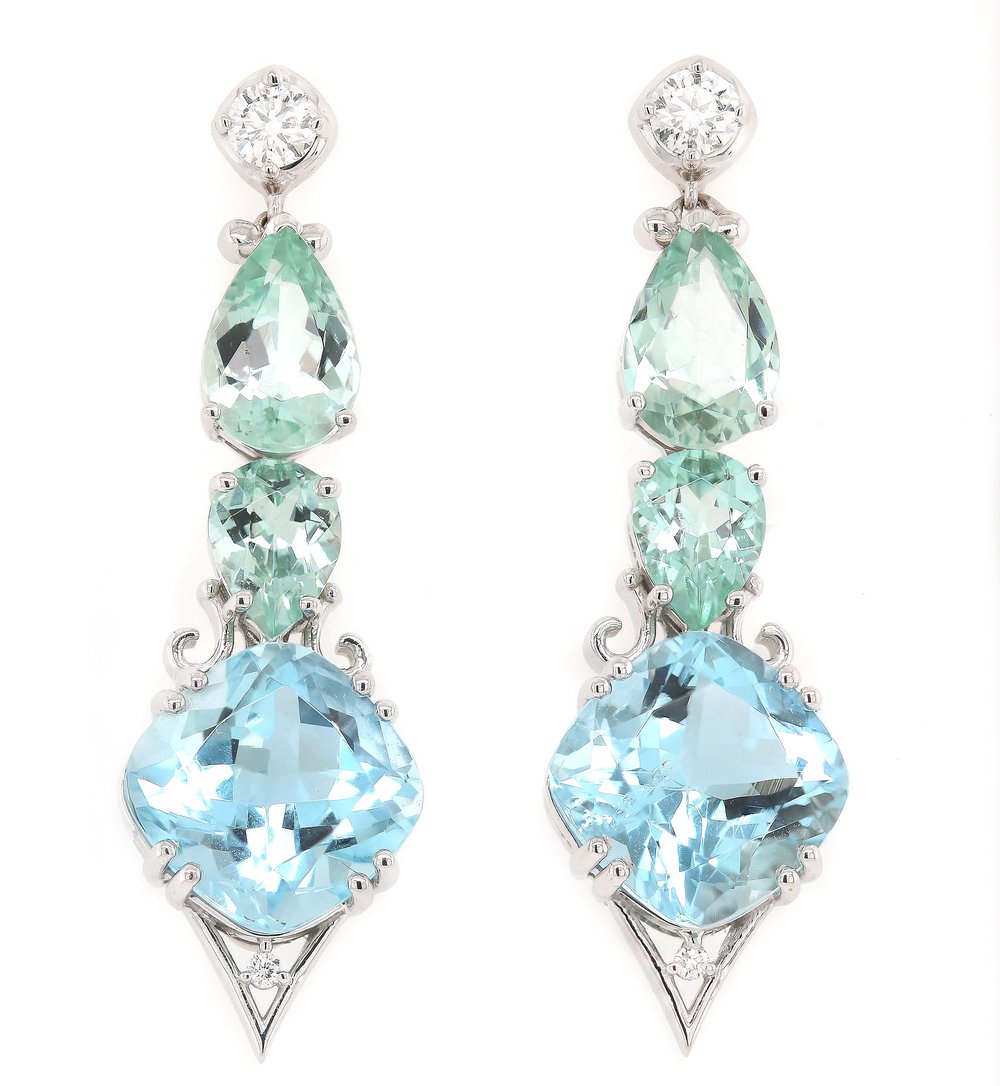This detailed image showcases a pair of intricate diamond earrings against a plain white background. At the very top of each earring is a small, circular white diamond, encased in a shiny silver prong setting. Descending from this, there is a light greenish-aqua teardrop-shaped diamond with its point facing up, set in the same reflective silver prong. Below this gem is another, smaller teardrop-shaped diamond of the same greenish-aqua hue, but with its point facing down. Further down, the earrings feature a large, almost circular, light bluish diamond, also encased in a detailed silver frame with several prongs holding it securely.

At the very bottom of the design, a silver piece extends downward to form a sharp, triangular point. Centrally placed within this triangle is a final, very small white diamond, held by three more prongs. The earrings are identical in every detail and are positioned side-by-side. The overall appearance of the gems and their intricate silver settings suggest a high level of craftsmanship, although the extreme close-up and absence of context make it difficult to determine the exact nature of the materials used or the scale of the earrings.